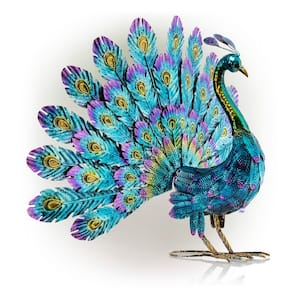Here's a detailed caption combining and refining the descriptions:

This image depicts a vibrant, artistic interpretation of a male peacock, with no border, artist signature, text, or watermark. Featured against a plain white background, the peacock stands about two feet tall with fully extended and elaborately detailed tail feathers. The body of the peacock is primarily blue, accented with patches of purple and green along the front. Its neck is adorned with striking yellow markings that extend up to its blue head, which features a yellow beak. The bird's feet and legs are yellow with black claws.

The peacock's tail feathers are an explosion of color, blending purples, blues, and yellows. The feathers are arranged in multiple rows, each adorned with pea-like dots that have yellow and black centers. At the base, the feathers are bluish, transitioning to purple at the tips. The central parts of the feathers boast yellow centers surrounded by bluish and purple hues, all unified through a striking interplay of vibrant colors. A subtle shadow beneath the peacock's feet grounds the image, adding depth to this colorful and exotic depiction.